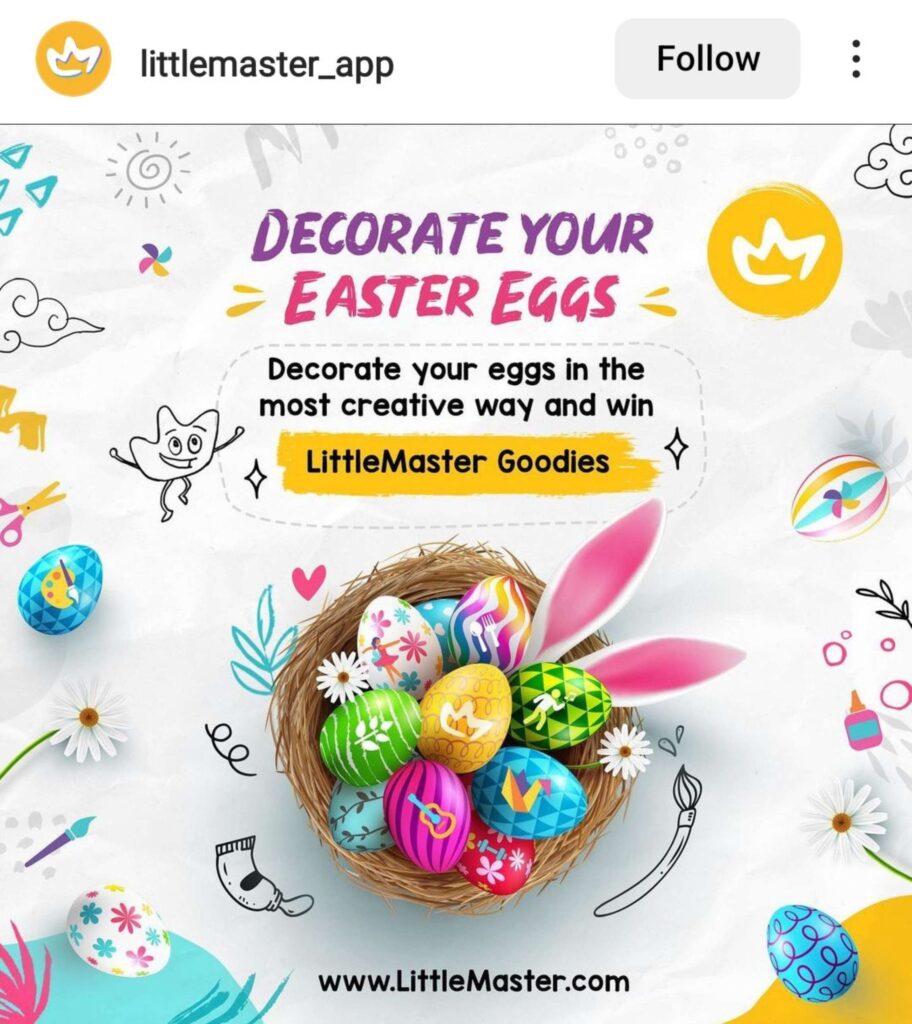In the top left corner of the image, the text "Little Master_App" is displayed. Adjacent to it on the right is a light gray follow button with the word "Follow" in black, and three vertically aligned dots, all set against a white background. An orange logo featuring a white, leaf-like element appears at the top, although its exact nature is unclear.

Below this section, the text reads, "Decorate your Easter eggs" and "Decorate your eggs in a most creative way and win Little Master goodies." This promotional message is centered above an overhead view of an Easter basket. The basket is woven from light brown material and contains an array of vibrantly colored eggs in shades of green, blue, purple, yellow, pink, orange, and red. Protruding from the basket are white bunny ears with pink inner linings. 

At the bottom of the image, the website URL "www.littlemaster.com" is provided. The entire scene is set against a white background embellished with small illustrations of paintbrushes, paint tubes, eggs, and leaves. Scattered around the basket are additional eggs that appear three-dimensional and realistic.

Additionally, various whimsical elements are included, such as a small, amoeba-shaped character with arms, legs, eyes, a mouth, and eyebrows, set against a backdrop interspersed with drawings of blue and yellow clouds and suns.